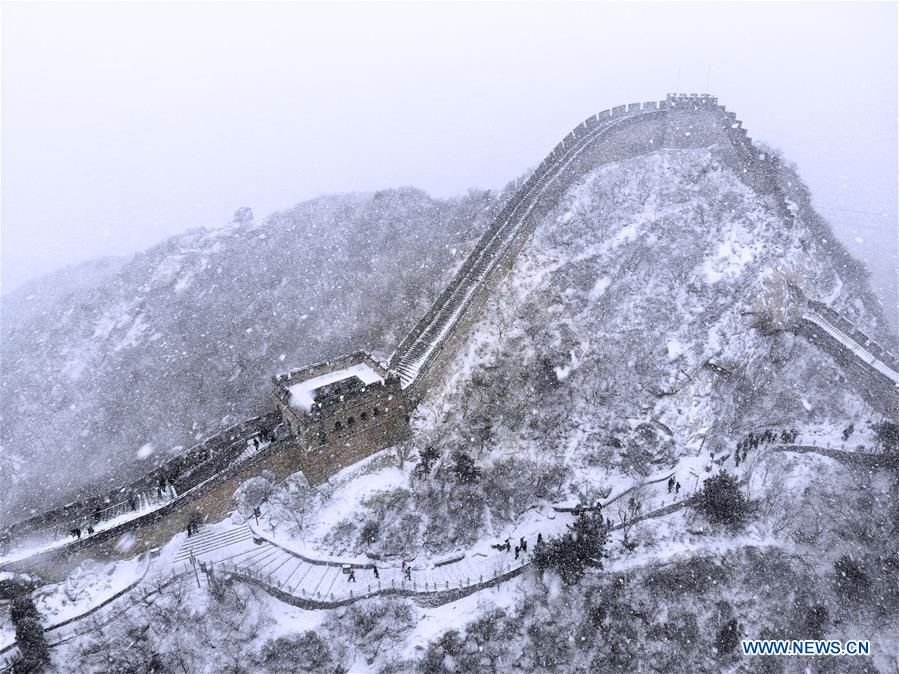This photograph captures a snowy day scene of the Great Wall of China extending up a large, snow-covered hill. Snow is falling gently, covering the ground, mountains, and the ancient wall itself. The sky is overcast and white, suggesting a snowstorm. At the bottom of the image, the text "www.news.cn" is displayed, indicating the source. The Great Wall ascends steeply up the hill, disappearing over the crest and reappearing on the other side. A brick building with four windows is visible along the wall. Numerous people are walking on the pathways, both along the Wall and on an adjacent, less steep route. The entire landscape is coated in a light dusting of snow, creating a picturesque winter scene.